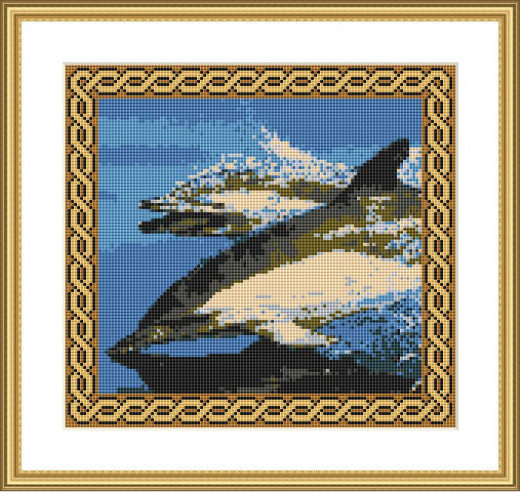This image portrays a framed digital artwork, likely created and rendered on a computer, of two dolphins swimming in the water. The frame is elaborate, featuring an exterior layer in brown, an interior layer in gold, and a double boundary with a white square border and a twisted, gold chain surrounding the central artwork. The focal point, the two dolphins, exhibits a low-resolution, pixelated quality, mimicking a stitched or mosaic-like appearance. The dolphins, identifiable by their characteristic noses, display a distinct contrast with white underbelly and black upper side, creating an almost orca-like appearance. This digital depiction is set within a dual-layered frame, suggesting a sophisticated and modern aesthetic suitable for any room in the house. The colors in the image include various shades of brown, gold, white, black, silver, and light blue, which contribute to the visual depth and intricate detailing of the artwork.